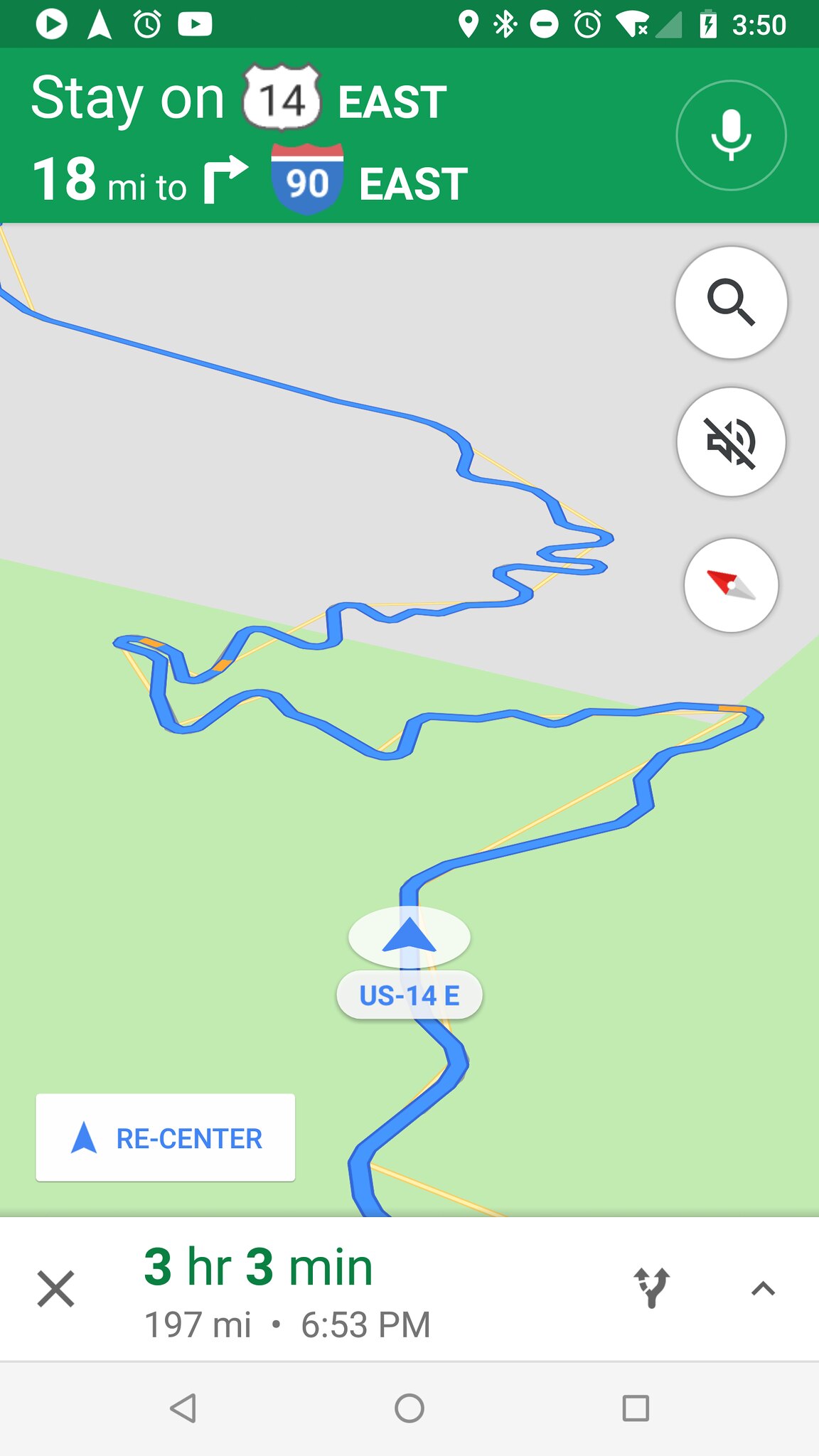This image appears to be a screenshot from a navigation app, possibly MapQuest or Waze, displayed on a smartphone, likely an iPhone. The top part of the screen shows typical phone indicators, including the time, signal strength, and battery life. Below that, the navigation instructions indicate to stay on Route 14 East for 18 miles until merging onto Route 90 East. The map visual depicts the outlined route in blue, traversing over a green background, which symbolizes terrain, and connecting to a gray background representing roads. It further indicates that the total trip duration is approximately 3 hours and 3 minutes, covering a distance of 197 miles, with an estimated arrival time of 6:53 PM.